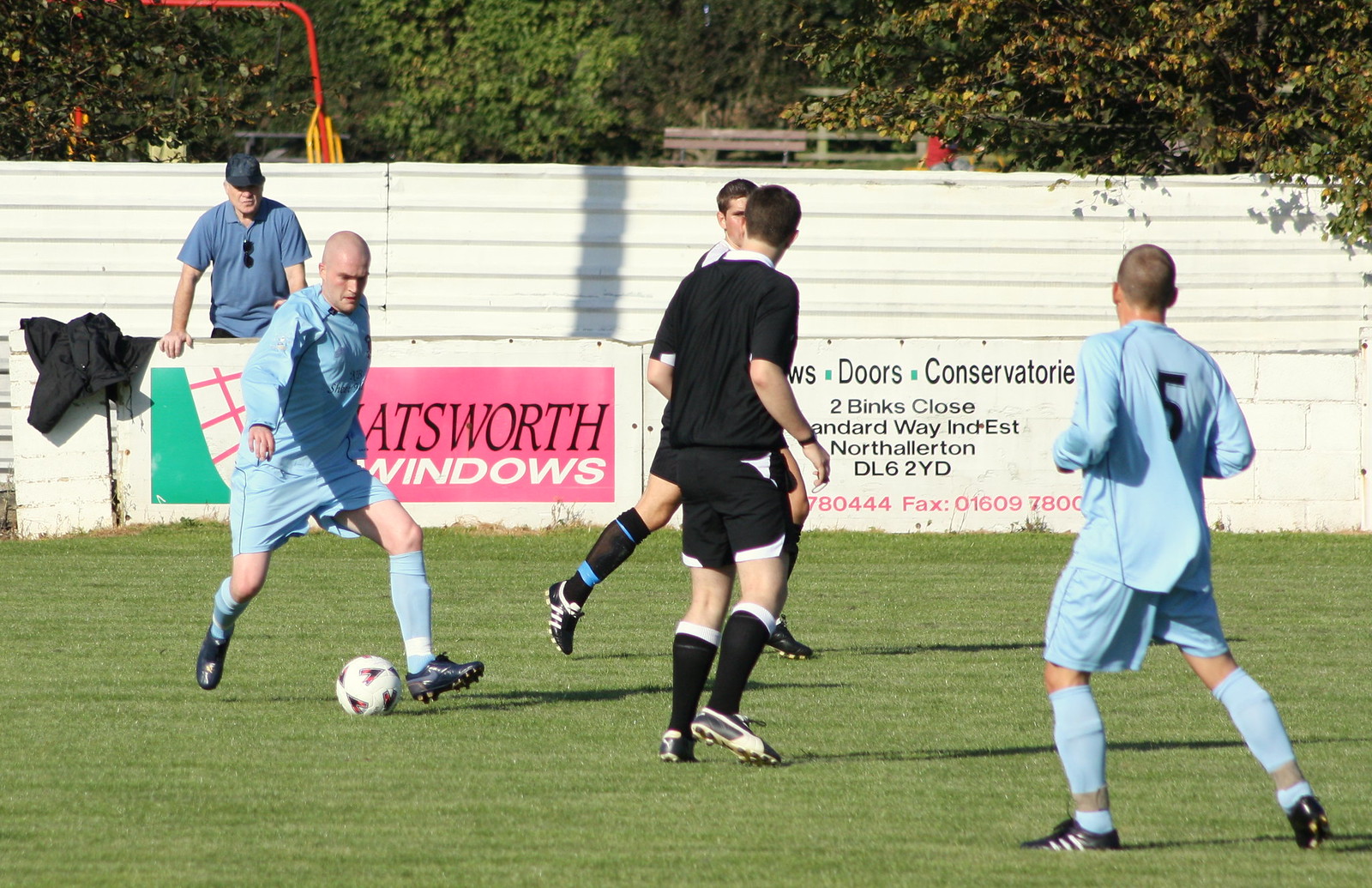In this sunny outdoor soccer game on a grassy field, the main focus is on a man in a sky-blue uniform—comprising a long-sleeved shirt, shorts, and socks—preparing to kick a white soccer ball. He appears to be bald and is wearing black cleats. Two men in black uniforms, consisting of a black top, shorts, socks, and sneakers with white elements, are positioned between him and another player in a matching sky-blue uniform on the right side of the image. In total, there are five visible players actively participating in the game. 

In the backdrop, a white wall or short cement fence with brick detailing is visible, adorned with various advertisements bearing partially legible text such as "ATS WRTH windows" and "Doors Conservatory 2." Behind this wall, tall metal fencing painted white and vibrant green trees with hanging leaves frame the scene. A spectator, dressed in a muted blue t-shirt and a hat, with sunglasses hanging from his chest, stands to the left side behind the fence. The bright sunny day enhances the vivacity of the scene, making the outdoor field appear particularly radiant and lively.